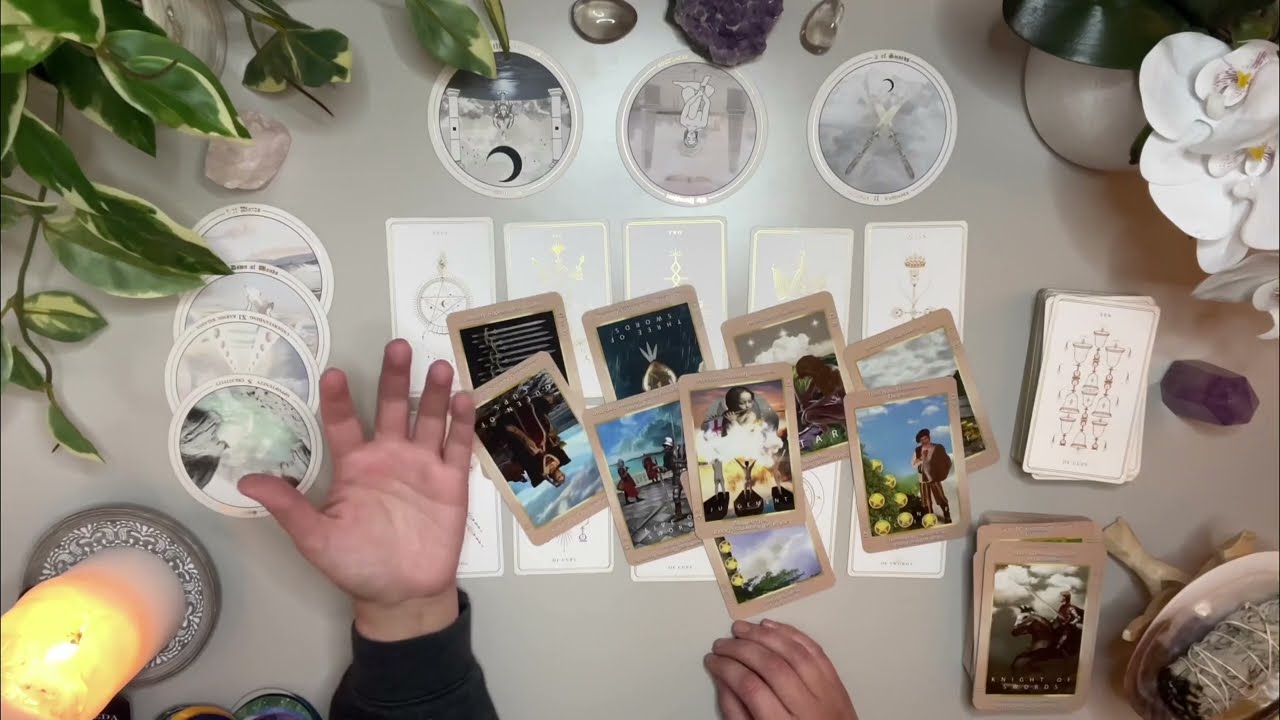This overhead photograph captures a meticulously arranged white table adorned with various objects. Centered on the table is an array of tarot-like cards, some faced upwards revealing images bordered in tan, and others faced downwards. To the right of these cards is a neatly stacked pile of similar cards alongside white flowers, a purple crystal, and a dish that might contain sage. Notably, there are circular objects, possibly CDs or coasters, featuring pastel colors. In the bottom portion of the image, a lit white candle sits on a round, brown, and white coaster in the bottom left corner. Nearby, a hand with a black sleeve is positioned palm-up towards the left side. The top left corner of the table is adorned with green leaves, presumably from a plant, and a white crystal placed in front of them. Munificent details such as these collectively create a scene rich with texture and intrigue.